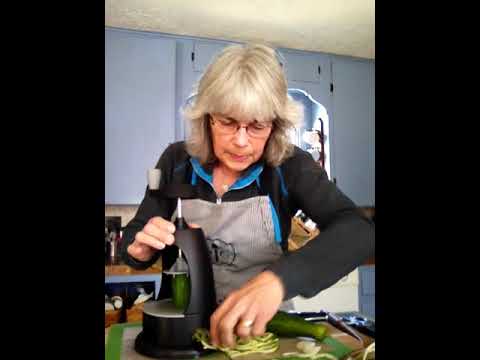In a cozy kitchen with gray cabinets and a blue wall, an elderly woman with shoulder-length, silver-gray hair and glasses is diligently slicing a cucumber using a black, rounded slicing machine. Clad in a long-sleeved black shirt and a black and light gray apron, she leans forward intently, her right hand steadying the machine while her left hand extracts the freshly cut green vegetable, now in thin, noodle-like strips, from the device. Above her, hanging cabinets provide storage, and the countertop behind her is adorned with various kitchen appliances, partially concealed by her right elbow. The entire scene is framed by thick black borders on the left and right sides of the image.